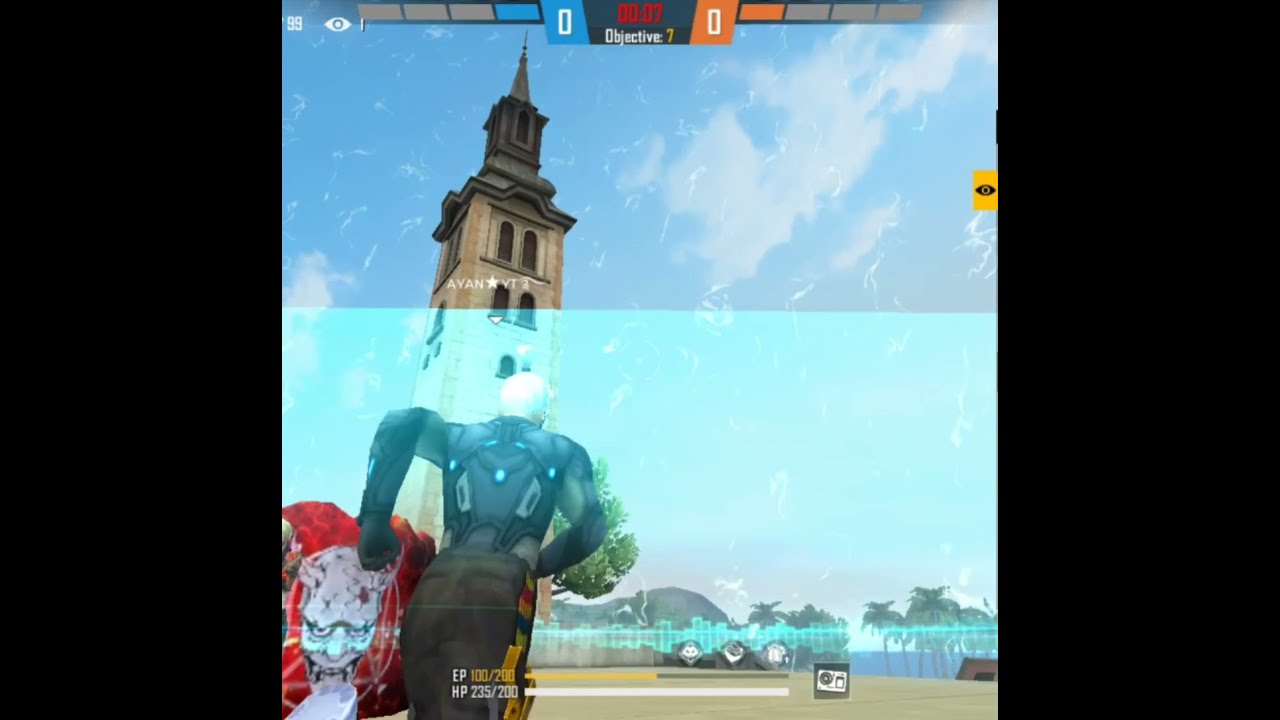This image is a highly detailed, partly computer-generated photograph resembling a screenshot from a video game. The central focus is on a scene set outdoors under a blue sky with white clouds. Dominating the middle of the image, a tall, narrow tower with a steeple leans slightly from left to right, creating a dynamic composition. A character in futuristic black armor with a white hat is depicted running across what appears to be a concrete or dirt lot, heading toward the tower. He is holding a red sign or blanket featuring a skull with horns and fangs. The background includes trees, the ocean, and various buildings and fences. 

Overlaying the tower image is a gaming interface. At the top, against a blue band, it reads "00:07," while an orange band displays "Objective 7" and "0." In the middle, the text "AYAN star VT" appears. The bottom of the image features player statistics, including "EP 100/200," "HP 235/200," and a heartbeat-like graphic. The lower left corner shows a menacing creature with a white body and horns, framed in red. Surrounding the central square image is a horizontal black border, enhancing the vividness of the colorful scene within.